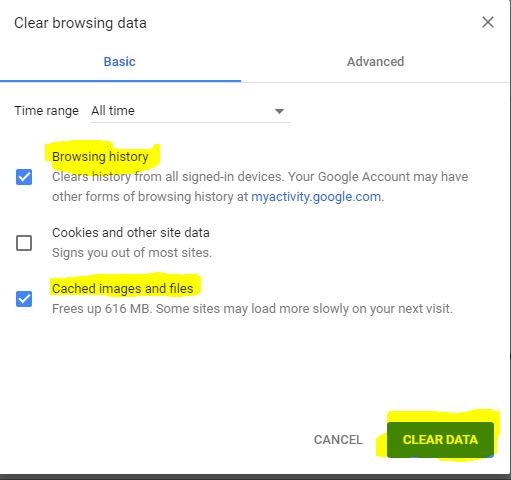The image depicts a computer screen showing the "Clear browsing data" settings in a web browser. The setting is open to the "Basic" tab, which is highlighted in blue along with an underline. Next to it, the "Advanced" tab is displayed in a lighter gray without any blue highlight. The primary section displays "Time range," set to "All time," with a downward arrow indicating the option to change the time range.

Three checkboxes are visible under this section. The first checkbox, labeled "Browsing history," is filled and highlighted with a yellow marker, extending slightly beyond the text boundaries. This option includes a note indicating that clearing history will remove it from all signed-in devices and mentions an alternative location for viewing browsing history, "myactivity.google.com," which is highlighted in blue.

The second checkbox, labeled "Cookies and other site data," is unchecked, with a note explaining that clearing this data will sign the user out of most sites.

The third checkbox, labeled "Cached images and files," is selected and highlighted with a yellow marker.

In the bottom corner of the window, there are two buttons: "Cancel" and "Clear data." The "Clear data" button is green and also highlighted in yellow, emphasizing the action button.

Overall, the image provides a clear view of the user's efforts to manage their browsing data, highlighting their selections and key features of the browser settings interface.